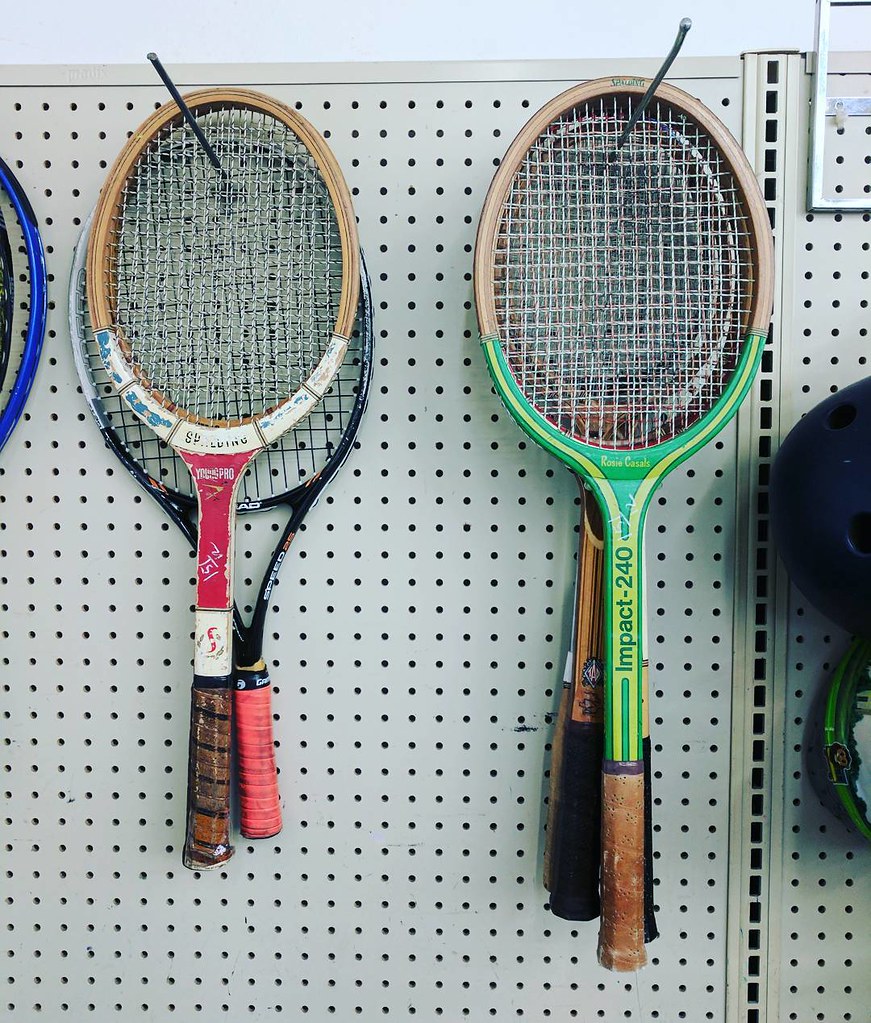This image captures a selection of six used, vintage-style tennis rackets displayed in a thrift store, likely a Goodwill, evidenced by the distinctive white perforated pegboard wall behind them. Each racket is suspended by its head on two long metal pegs. The pegboard, characteristic of retail display setups, features numerous small holes for versatile item arrangement. The rackets, showcasing wear and tear, have diverse designs and colors. On the right peg, the foremost tennis racket is painted green with yellow stripes and has a dark brown handle, accompanied by three other similarly-sized wooden rackets mostly obscured from view. The left peg holds two rackets, with the front one painted red with a white hoop and a brown handle, while the rear one appears smaller, possibly for racquetball. The image's framing includes an additional partial view of a blue racket on the left and an indistinct black object on the right, adding to the sense of a cluttered, second-hand store setting.